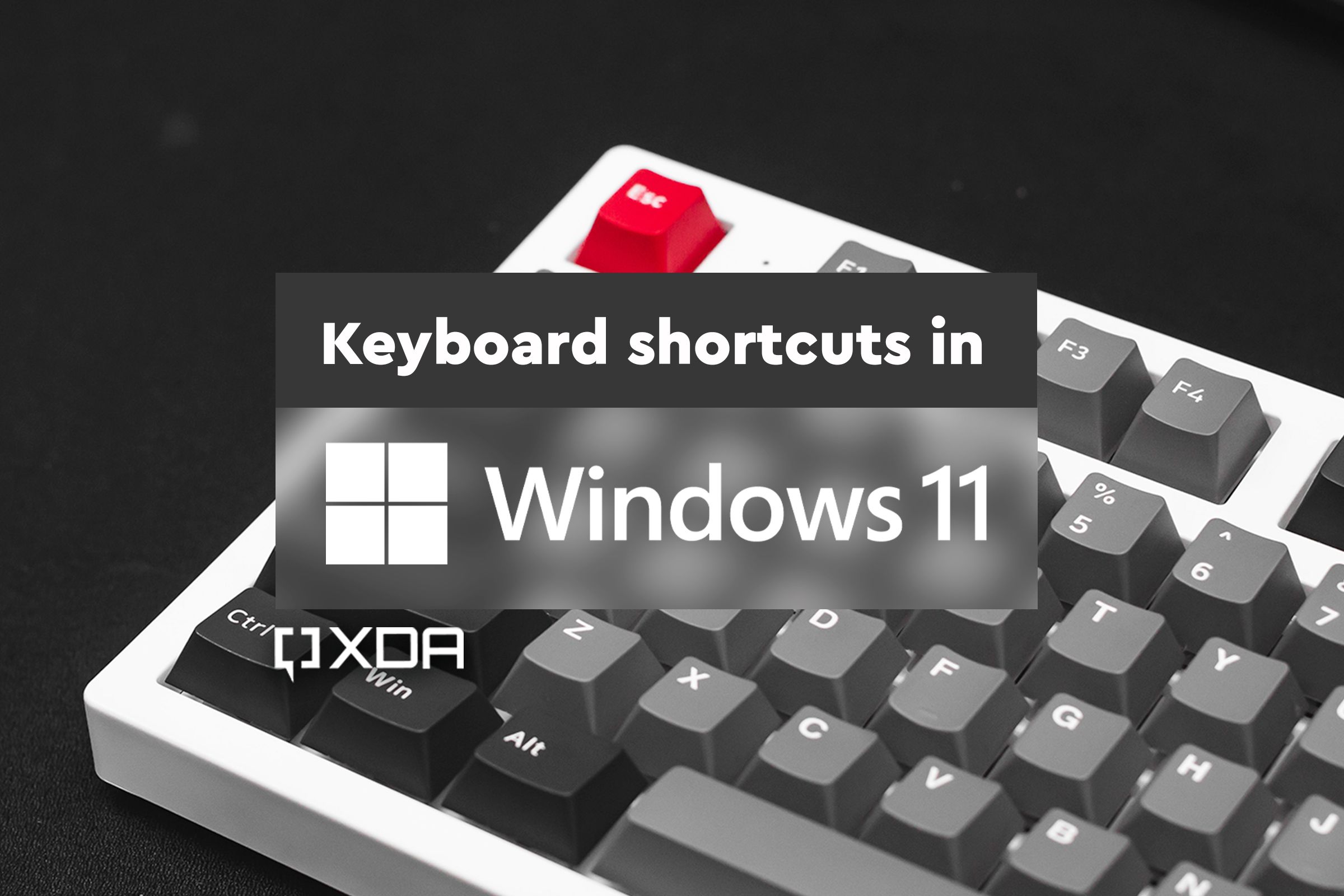The image shows a partially visible white keyboard turned at an angle, with keys primarily in black and dark gray. The escape key, located at the upper left-hand corner, is a distinctive bright red. The keyboard features white font labeling the letters, numbers, and command keys. It is set against a dark matte background. Overlaid at the top is a title in a dark gray band that reads "Keyboard shortcuts in Windows 11". Adjacent to this title is a square Windows 11 logo comprised of four squares. Below the title, there is a transparent, blurred section obscuring part of the view. The keyboard’s visible keys do not extend beyond the 7 and J keys in the standard QWERTY layout. At the bottom of the title, ambiguous text resembling "OXDA" or "QXDA" appears.